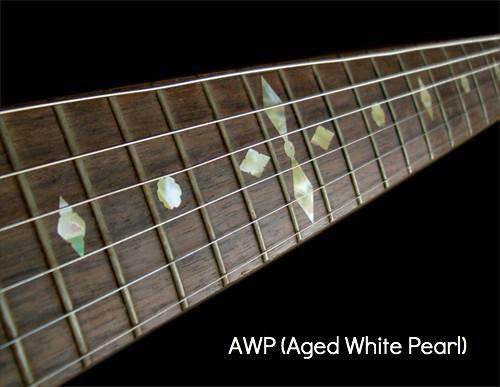This is a detailed photograph of a wooden guitar neck, featuring a dark brown hue and six silvery strings stretched across its length. The background is completely black, isolating the neck and making it the focal point of the image. The neck is adorned with several gold embellishments between the divots where the strings rest, including a clover-shaped design and two diamond-shaped ones. In the lower right corner, white text reads "AWP" with "Aged White Pearl" in parentheses, likely referring to the decorative patterns on the neck.